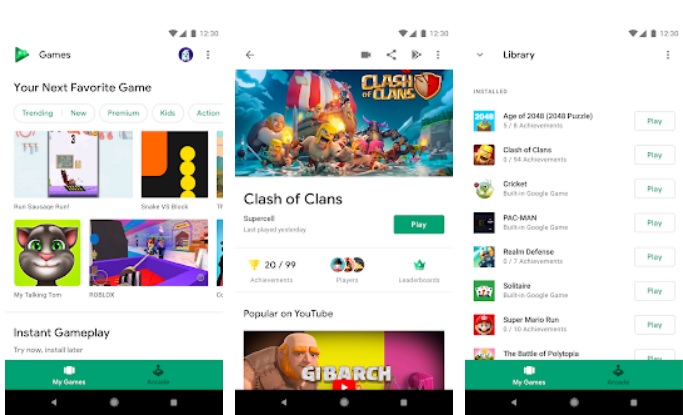This image features three side-by-side screenshots from the Google Play Store, showing different sections of the app. 

**Left Panel:**
The left screenshot highlights the "Games" section of the Play Store, which is marked by an icon of a game controller over a triangle at the top. The heading "Your next favorite game" introduces various categories such as "Trendy," "New," "Premium," "Kids," and "Action." Beneath these headers are several game icons and titles, including "Snake" and "My Talking Tom," but some titles are unreadable. The footer features "Instant Gameplay," with a green background, followed by the navigation bar.

**Center Panel:**
The center screenshot showcases the game "Clash of Clans" by Supercell. A visually appealing graphic spans the width of the panel. Just below the graphic, the game's title, accompanied by a "Play" button indicating the game is already installed, is prominently displayed. It shows 20 out of 99 achievements have been unlocked, and a leaderboard with various players is shown below. Further down, there's a section titled "Popular on YouTube," followed by the navigation menu at the bottom.

**Right Panel:**
The right screenshot shows the "Library" section, displaying an array of games installed on the user's device. Visible titles include "Age of 2048," "Clash of Clans," "Cricket," "Pac-Man," "Realm Defense," "Solitaire," "Super Mario Run," and a partially legible title, possibly "Battle of Polyopolis." Each game has a "Play" button next to it. Adjacent to this section is an "Arcade" tab. The footer repeating the navigation menu is shown at the bottom.

Note: The screenshots are quite blurry, making some text difficult to read clearly.